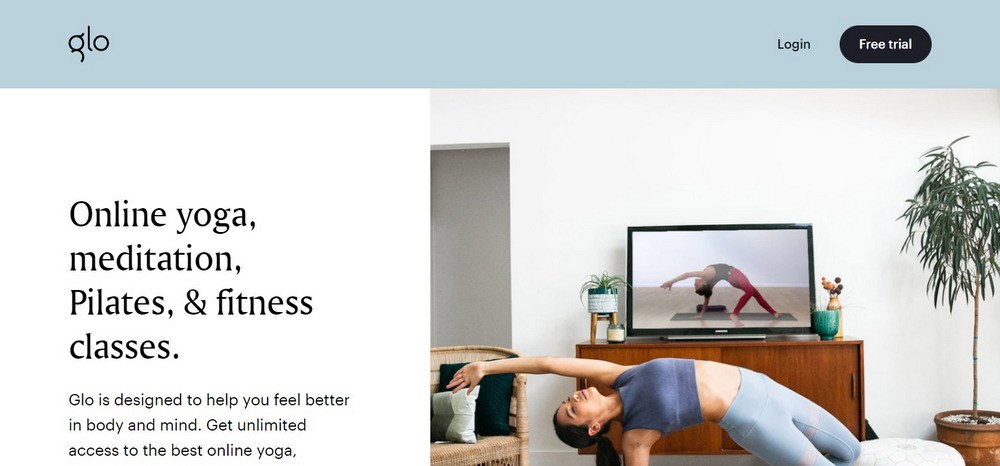A vibrant image promoting Glow, an online platform for yoga, meditation, Pilates, and fitness classes. The focus is on a woman with a black ponytail, dressed in blue yoga pants and a coordinating dark and light blue sports bra. She is performing a dramatic yoga pose, resembling a rainbow with one hand reaching for the sky and the other grounded on the floor. In the cozy setting, complete with a chair adorned with pillows and a verdant plant, she mirrors the instructor's pose displayed on the TV in the background. The black oval frame amplifies the elegance of the scene, while text highlights Glow's offering of free trials and unlimited access to premium online yoga content, designed to enhance both body and mind.